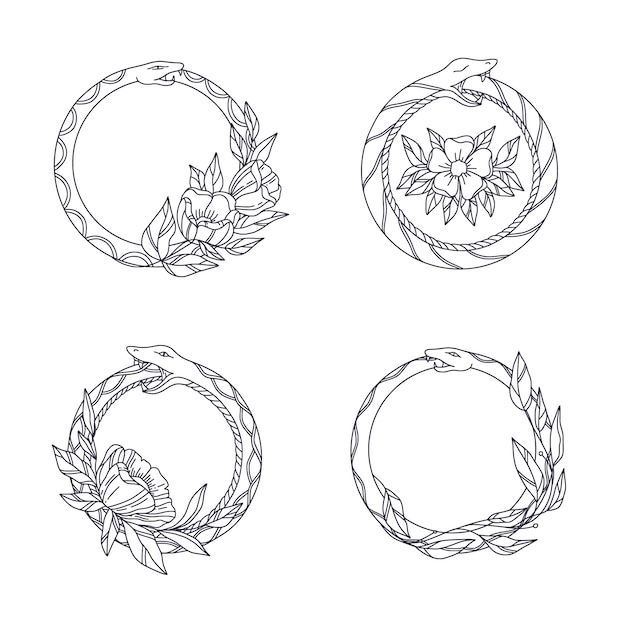The black-and-white image features four distinct Ouroboros designs, each depicting a snake swallowing its own tail, arranged in a row of two at the top and two at the bottom. Each snake forms a circular wreath with intricate details. The top left Ouroboros has a beveled or hump-like pattern with round shapes on its back and flowers situated at the bottom right of the circle. The top right Ouroboros has a striped pattern and a large five-petaled flower with surrounding leaves in the center of the ring. Both top snakes face towards the right.

In the bottom row, the left Ouroboros shows a similarly beveled or hump-like design with oval or teardrop shapes and flowers located at the bottom left. The snake's head also faces left. The bottom right Ouroboros features stripes with leaf-like shapes and leaves growing from the bottom right of the ring, with the snake's mouth closed tightly and head facing the left side, distinctly lacking any flowers in its design. All snakes exhibit a double border pattern on their bodies, enhancing the detailed nature of the artwork.